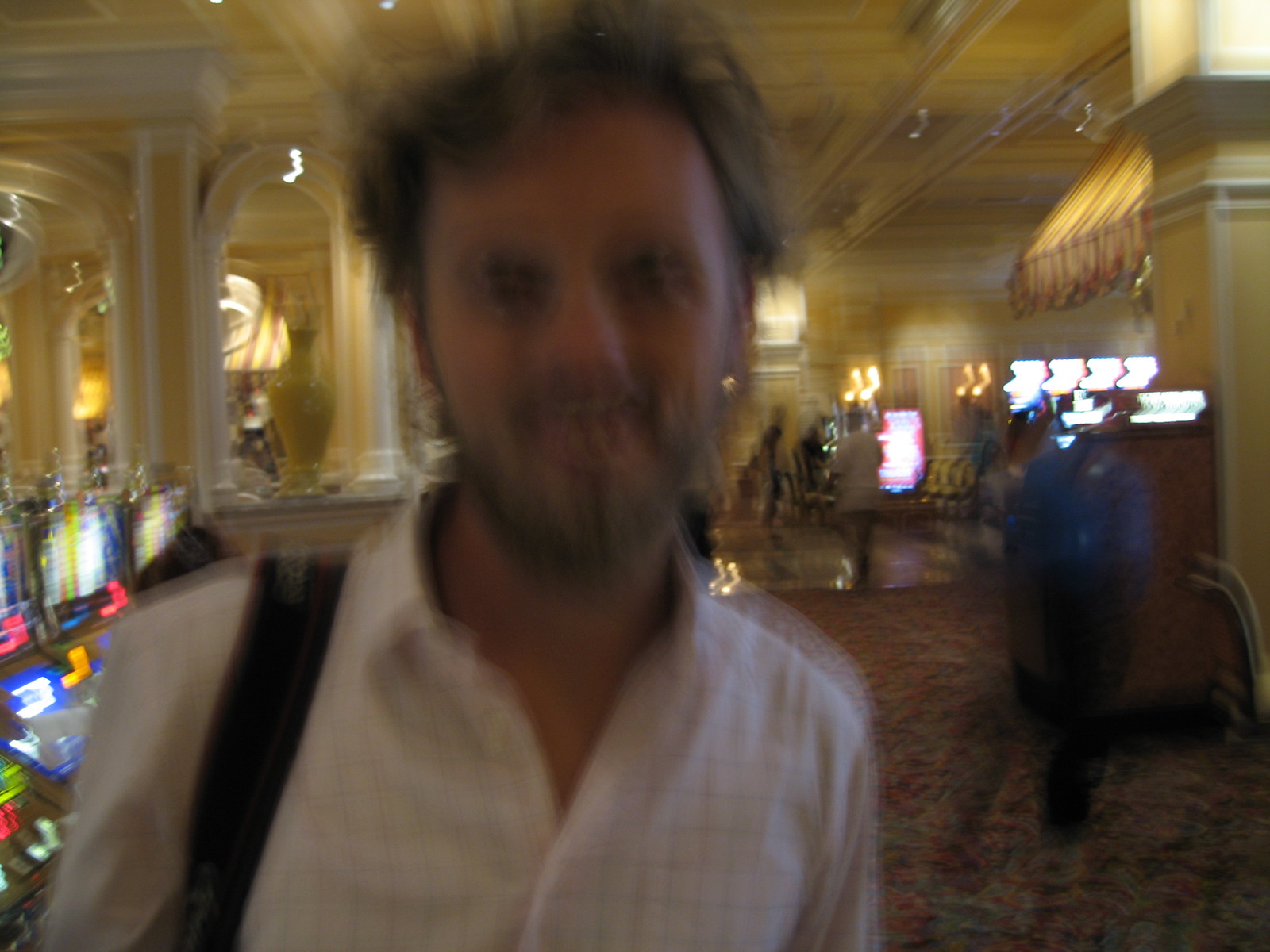The image captures a man in a heavily blurred setting that appears to be a casino, marked by its intricate yellow walls, multiple archways with lighting, and prominent columns. The man, who is the main focus, has light brown hair that is slightly disheveled, a beard, and a mustache. He's wearing a white button-up shirt with a blue square pattern, and the top few buttons are undone. A black backpack strap, which features white lines and some indistinct lettering, is slung over his right shoulder. Although the photo is blurry, you can tell he is sticking out his tongue and smiling. In the background, you can discern brightly lit slot machines showing vibrant colors like pink, orange, and blue, as well as other blurred figures, including a man in a gray suit coat walking away.